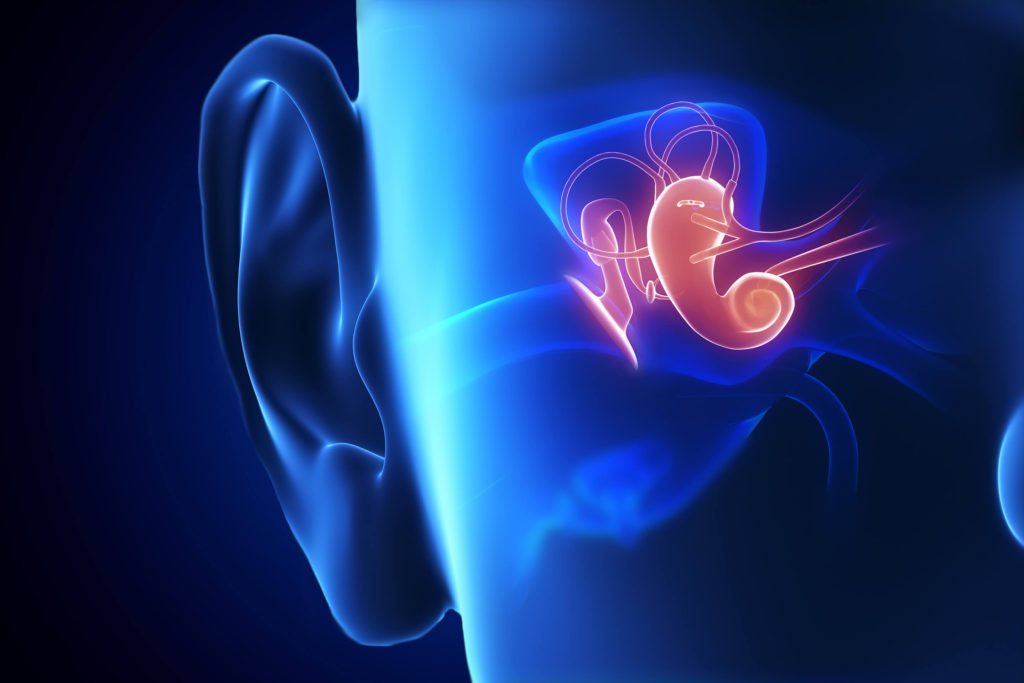The image is a computer-generated, scientific representation showcasing the detailed inner workings of a human ear within a transparent blue head. The primary focus is on the right ear, visible from the side, revealing the intricate pathways connecting the outer ear to the inner ear. The transparent blue head allows a clear view of these pathways, with the ear structures depicted in a detailed, almost 3D model format. The eardrum stands out prominently, glowing orange to highlight its presence amid the otherwise blue structures. The inner ear canals appear as curling tubes, creating a complex network, while the earlobe and external portion of the ear are also visible. The majority of the image maintains a transparent blue appearance, which contrasts with the bright orange eardrum, providing a stark and educational illustration of the ear's anatomy.